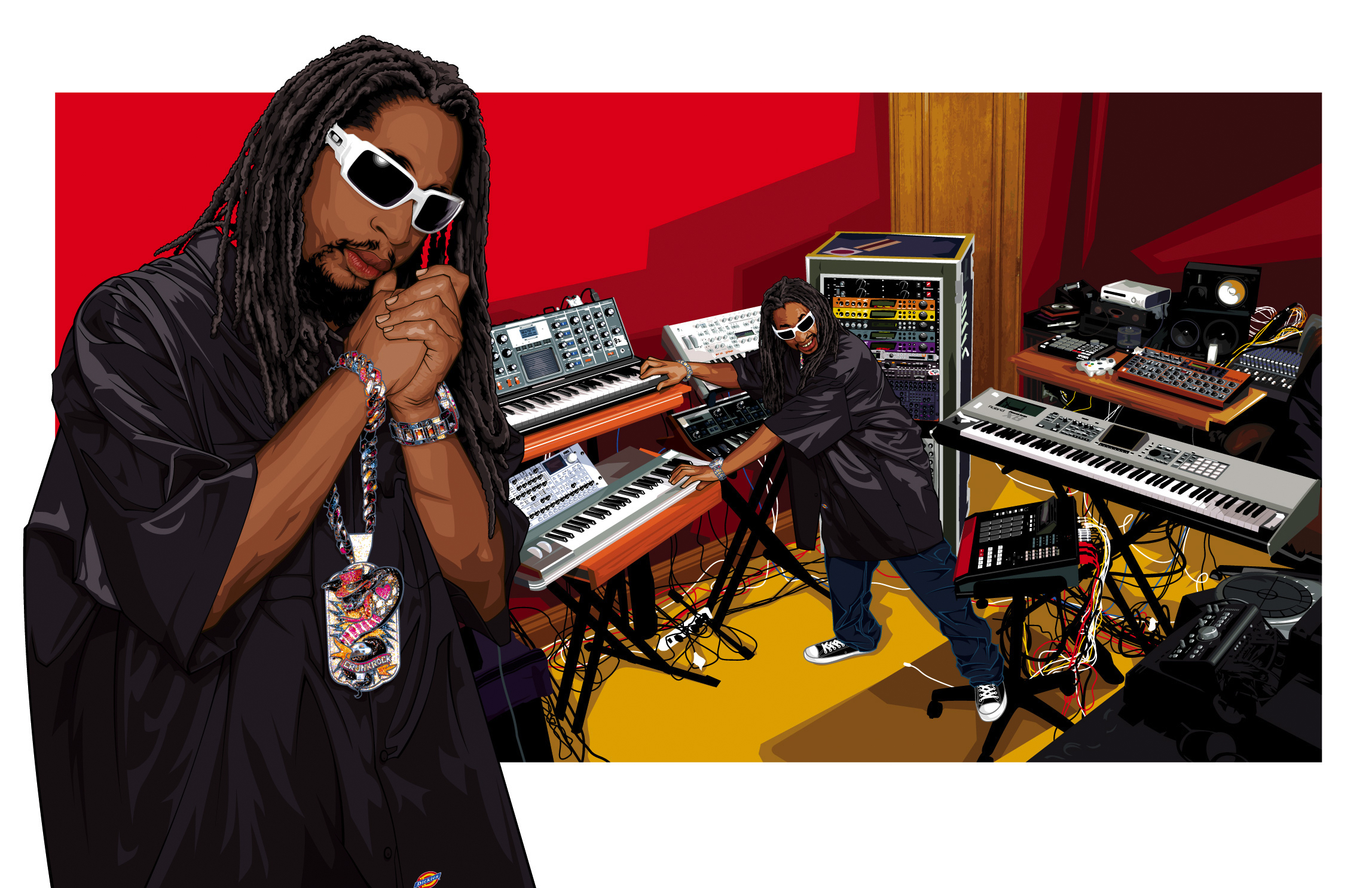This composite drawing prominently features rapper Lil Jon. On the left side, a large graphic of Lil Jon depicts him with long black dreads, white sunglasses, and a black baggy shirt adorned with a substantial necklace, bracelet, watch, and black shoes. His hands are clasped together. The backdrop showcases a vibrant red wall and yellow floor. To the right, a smaller depiction of Lil Jon, in the same attire, is seen energetically making music in a studio filled with various keyboards, synthesizers, drum pads, and other music equipment, exuding a sense of creative enthusiasm.